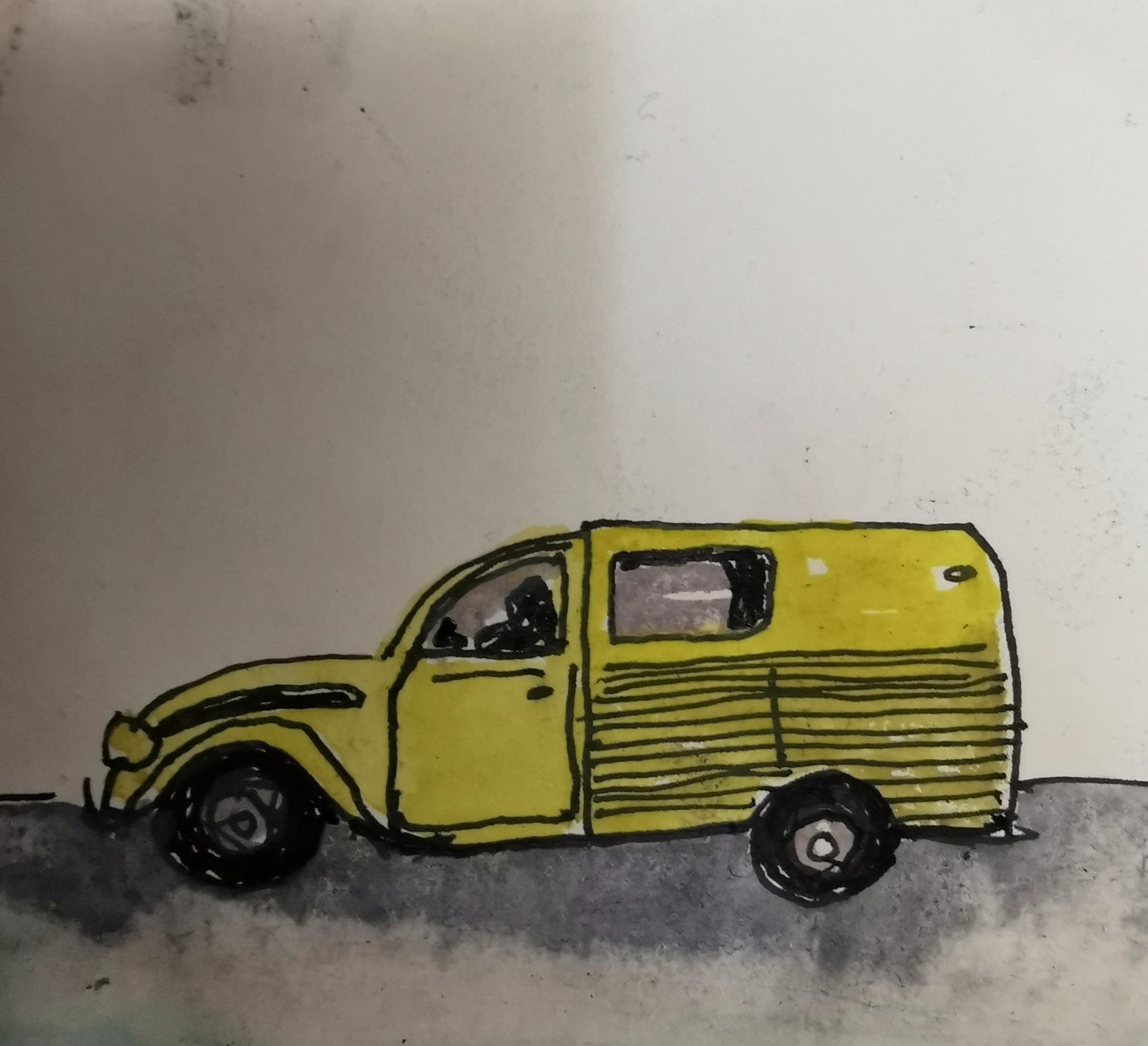The image is a color drawing on white paper, depicting an old-fashioned yellow truck or bus with black tires. The vehicle, drawn using simple, child-like strokes, features a back compartment with black horizontal lines and a small window for passengers. The front of the truck has yellow headlights and another window, with a possible depiction of a person inside. The truck casts a shadow on a gray asphalt-like ground, transitioning from a lighter gray at the bottom to a darker gray towards the top. Above the truck, the background remains white with random little black markings in the upper left-hand corner. The tires also have silver and white circles in their centers, enhancing the detailed yet whimsical rendering of the vehicle.